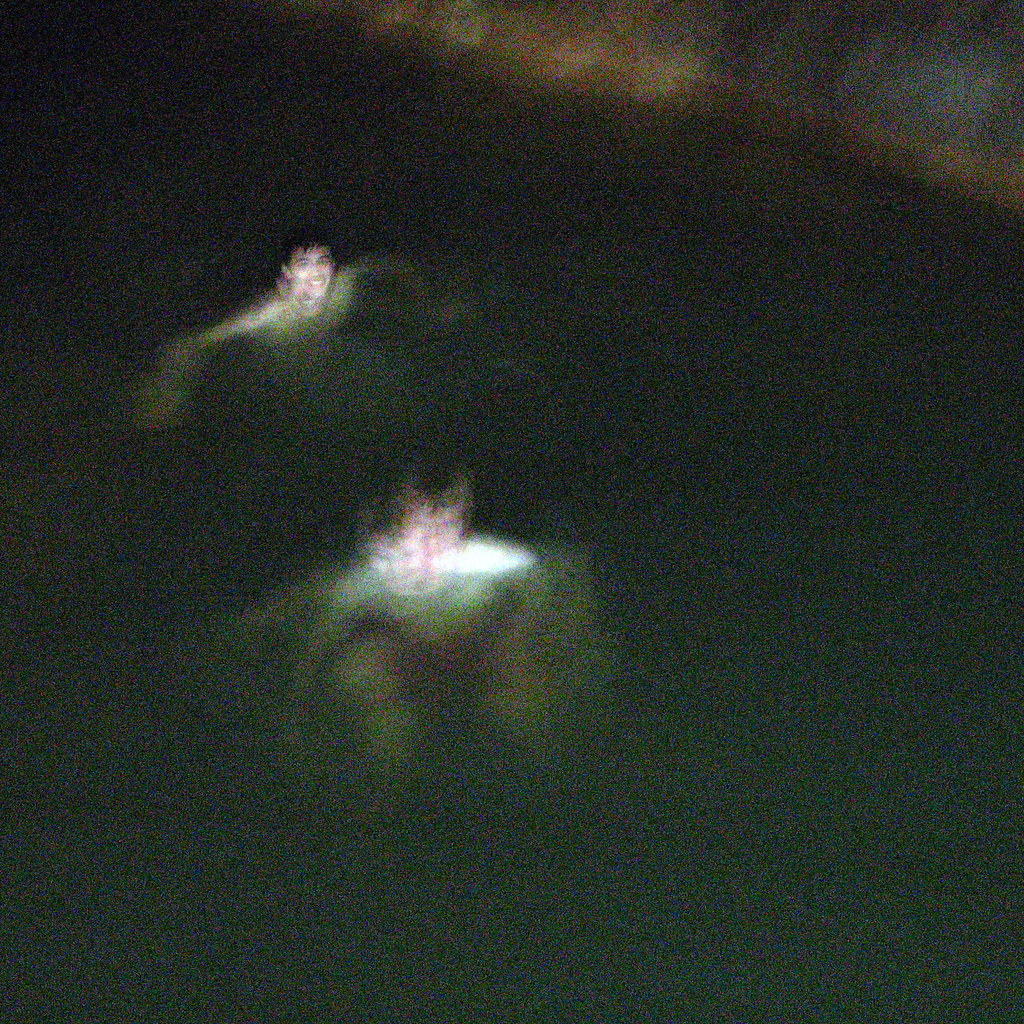In this out-of-focus, seemingly double-exposed photograph, two boys or young men are seen swimming in a dark, possibly natural body of water, resembling a swimming hole. The water appears almost black, adding a dramatic contrast to the scene. 

The boy in the back is positioned towards the upper left corner of the image. His face appears twice, suggesting a reflection or a result of multiple exposures. He has dark hair, dark eyes, and dark eyebrows, and he is smiling while looking directly at the camera. His arms are outstretched, as if treading water.

In the middle of the photo, another boy with lighter brown hair is visible. His face also seems to be duplicated, with one image facing straight ahead and the other seemingly looking down towards the water. His shoulder appears white, standing out against the dark water.

The bank of the swimming hole is visible in the upper right-hand corner, hinting at the serene yet somewhat mysterious setting of this moment.